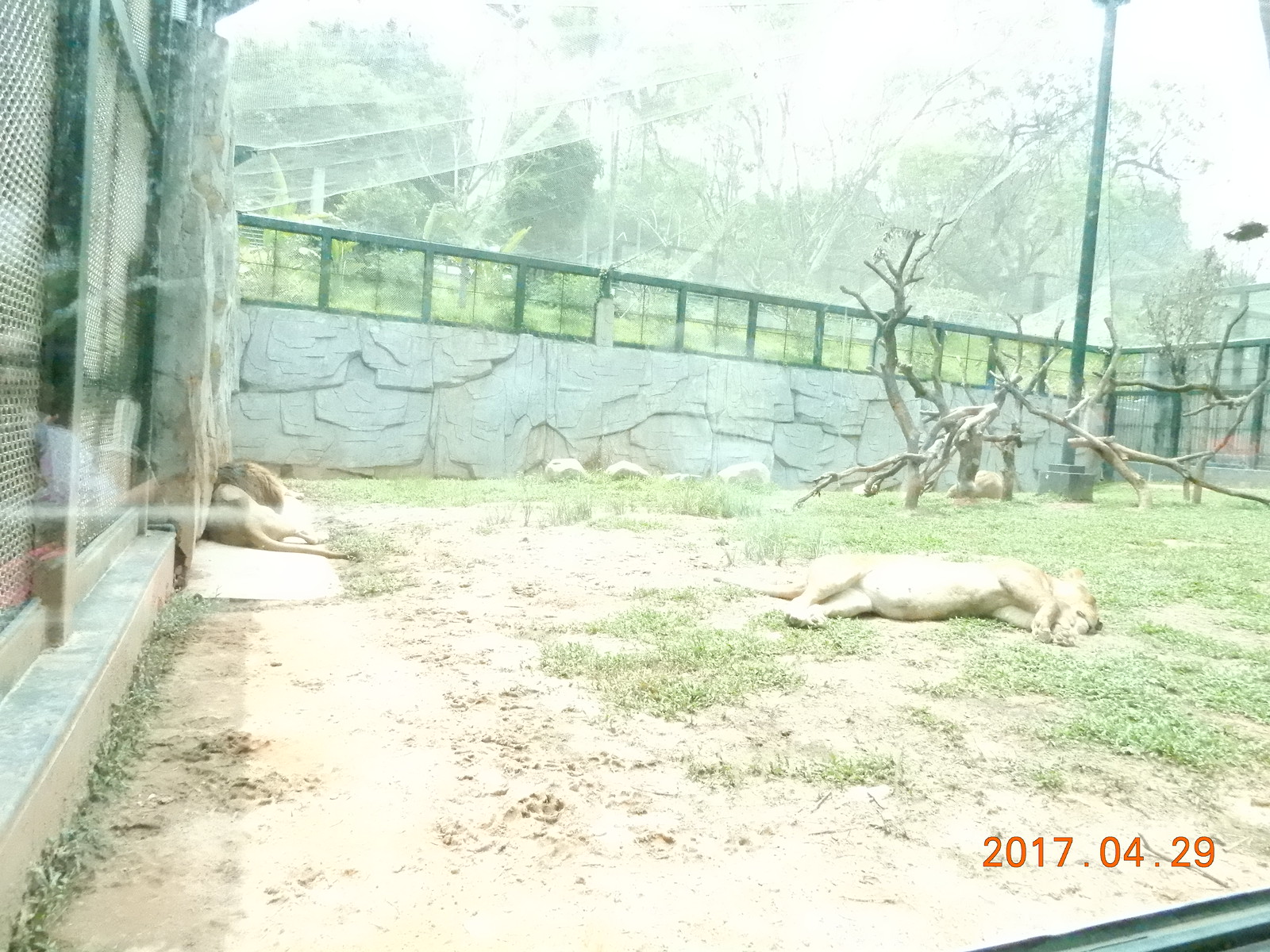This faded, older photograph, captured through glass or plastic, depicts a zoo enclosure from what seems to be a below-ground-level viewpoint. The image shows two lions resting in a sunlit area, though the overall scene is somewhat grayed and blurred. The enclosure features a combination of gray, stone-textured walls and a green-framed glass railing. The floor is divided into a white-brown dirt section on the left and a grassy area on the right. One lion, with a distinctive mane, is lying against the left wall, while the other, mane-less, is sprawled in the middle, belly up. In the backdrop, there is a dead tree with branches strewn across the ground, and a tall metal pole, resembling a street lamp, extends beyond the frame. The entire enclosure seems to be covered with a net or screen. Faintly visible in the lower right-hand corner is a watermark with the date "2017-04-29."